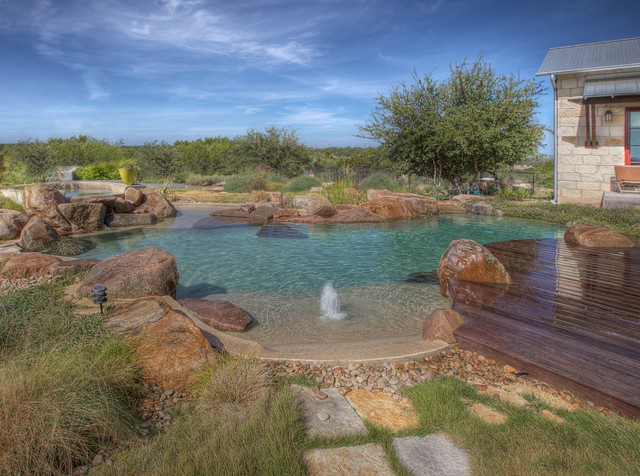The image depicts a tranquil backyard scene centered around a custom-made, bean-shaped teal pool. The pool's exterior is lined with pebbles and large decorative brown boulders. At its center, a fountain spout creates a small tuft of white water, adding to the serene atmosphere. On the right side, a rustic wooden deck with a shiny, brown-brandy finish extends from a light beige or white brick ranch-style house. A stone pathway, embedded in the grass, leads from the deck to the pool area. The backdrop features lush greenery, including a large bush and surrounding trees, under a vivid blue sky adorned with wispy clouds. A lone lawn light is visible at the bottom left corner, indicating that the photograph was taken during the daytime.